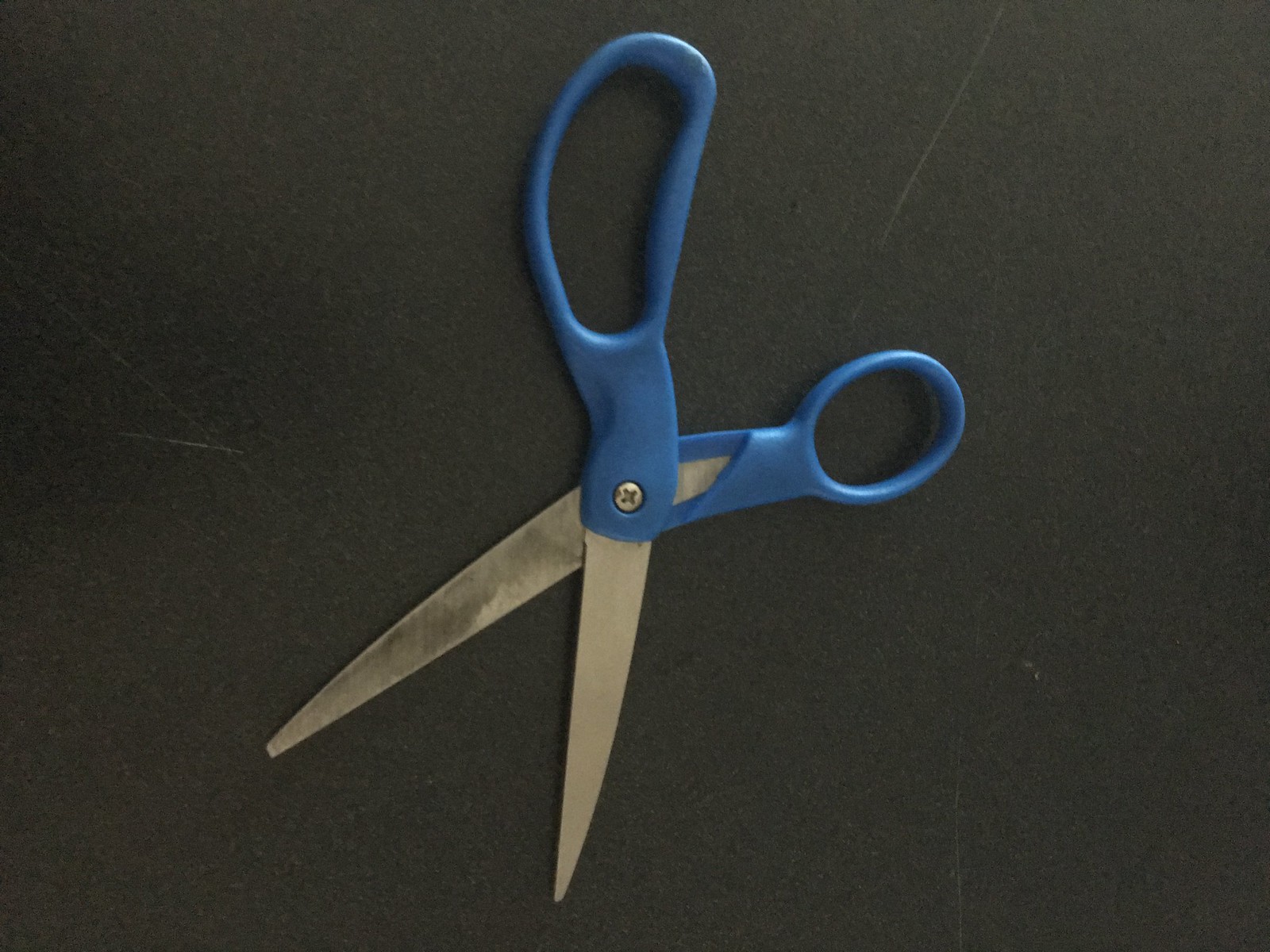This landscape-oriented photograph showcases a well-used pair of adult-sized scissors positioned horizontally. The background appears to be a dark gray or black surface, possibly a table or a piece of black paper, marked with a few white, hairline scratches. The scissors, featuring blue plastic handles - one oval for the fingers and one more circular for the thumb - are open at approximately a 30-degree angle. The stainless steel blades are prominently visible: the top blade, clean and pointing downward, contrasts sharply with the bottom left blade, which shows signs of use with dark gray smudges and tarnish. A central screw holds the blades together, hinting at the pair’s long history of use.